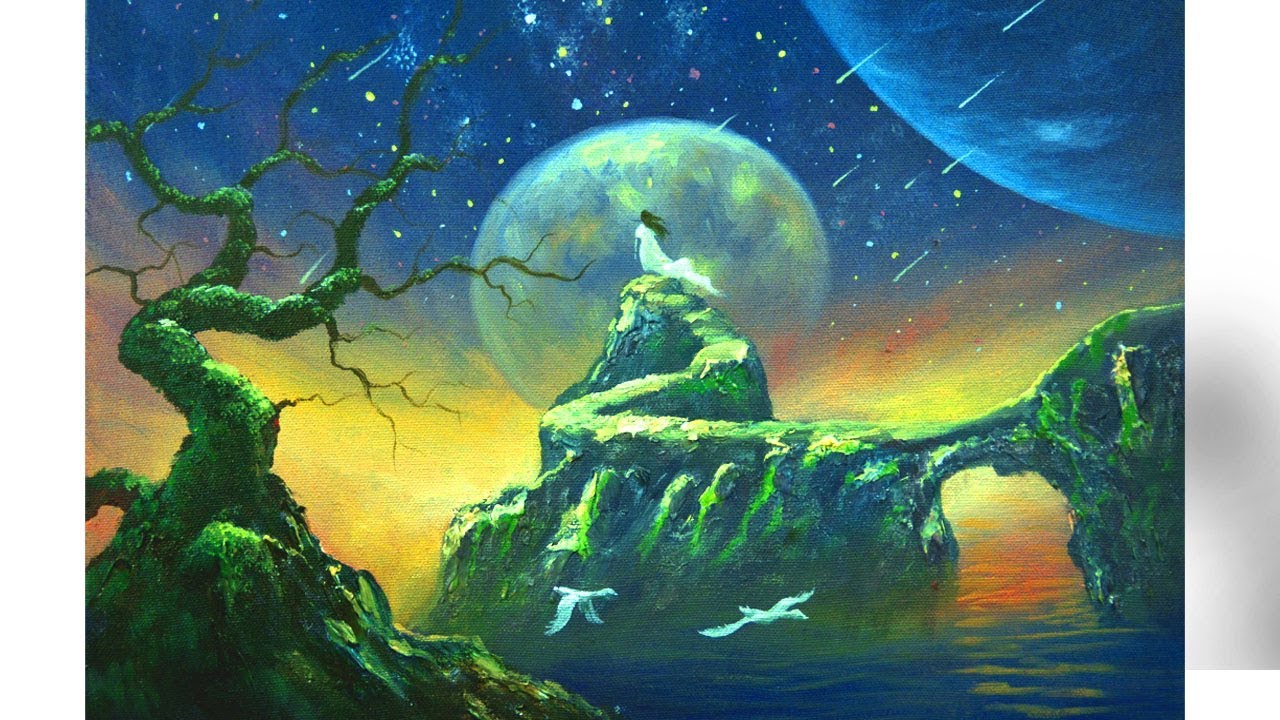This painting captures a serene yet otherworldly scene centered on a woman with long brown hair, seen from the back, adorned in a flowing white dress. She stands on a stone pathway that snakes upward and outward, eventually leading to a small natural bridge interlocking with another part of the pathway that extends off-screen to the left. Beneath this path and bridge, we see water, indicative of a lagoon-like area surrounded by rocky outcrops. On the far left, a dead tree emerges from the rocky terrain. The sky above is dominated by a large, metallic-looking planet in front of the woman, alongside another sizable, blue-hued planet in the top right corner. The backdrop features a blend of oranges and yellows at the horizon, transitioning into a rich, star-filled blue sky, with yellow stars and white streaks of shooting stars or comets illuminating the scene. Additionally, a few birds are seen flying in the sky, adding life to the tranquil yet mystical atmosphere.